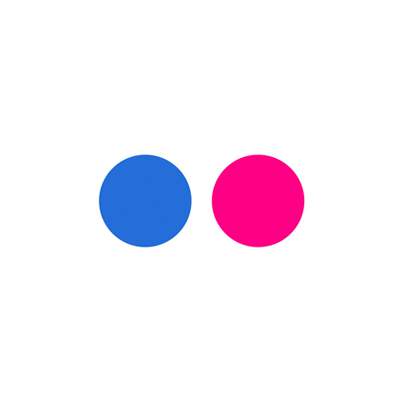The image depicts two large, solid-colored circles, each approximately an inch in diameter, set against a white background. One circle is in a vibrant royal blue, and the other is in a striking hot pink. These colors, while both bold, are harmoniously complementary and create a visually appealing contrast. Positioned side by side, the circles evoke a playful resemblance to the eyes of a cartoon character. The image, simple yet expressive, highlights the vivid hues of royal blue and hot pink, colors often favored in fashion for their strong, positive impact.